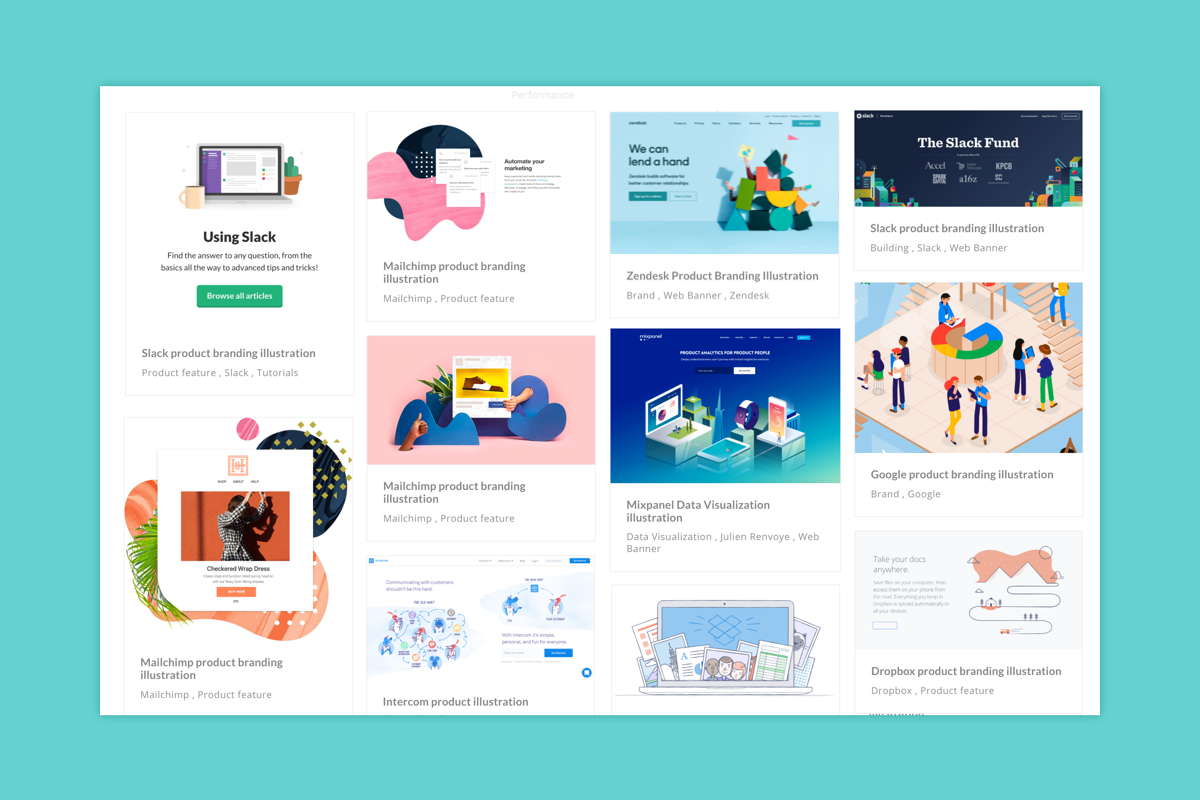A detailed and thoroughly cleaned-up caption for the described image is:

"This is a screenshot of a web page displayed on a teal background. The rectangular web page showcases a total of 11 options, each accompanied by distinct illustrations. The first option, titled 'Using Slack,' features a drawing of a computer and includes a prompt to 'Browse all articles.' The second option presents abstract art and is labeled 'MailChimp Product Branding.' Following this is 'Zendesk Product Branding Illustration,' featuring another unique image.

The fourth listing, 'Slack Fund,' is succeeded by another 'MailChimp Product Branding Illustration,' depicting a different illustration. Then there's 'Mixpanel Data Visualization Illustration,' followed by 'Google Product Branding Illustration,' which includes the iconic, multi-colored 'G' of Google surrounded by small drawings of people walking around and ascending stairs.

Further down, there's an ad for 'Dropbox Product Branding Illustration,' promoting a 'Dropbox Product Feature' and depicting a computer with papers surrounding it. Another 'MailChimp Product Branding Illustration' shows a lady dancing. The final entry, 'Intercom Product Illustration,' is distinguished by various colorful icons in red, blue, yellow, and green hues."